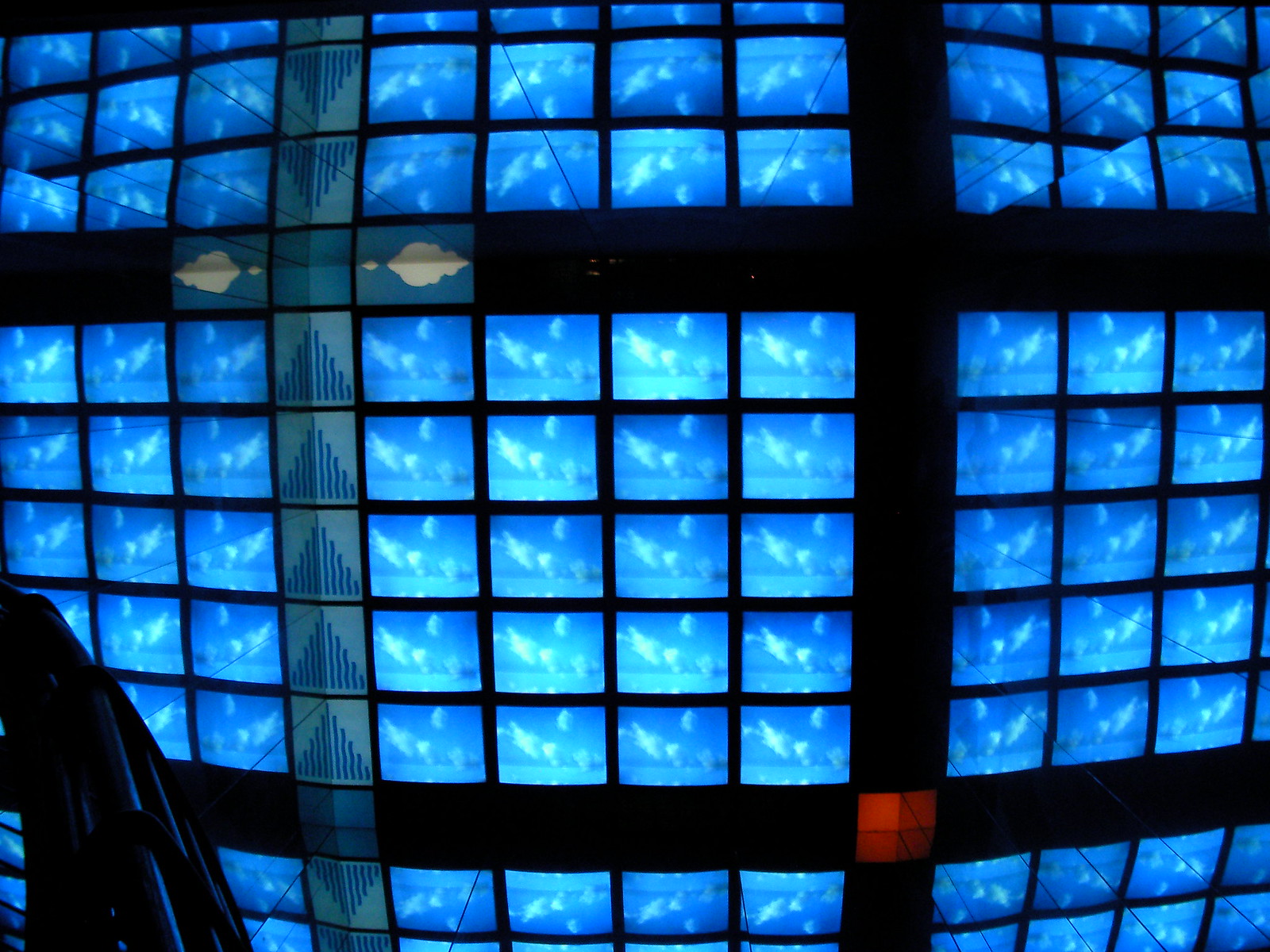The image depicts a large wall fully covered with over 50 small TV screens, each displaying the same aquatic scene featuring blue skies, white clouds, and a body of water with possible marine life, such as dolphins. The screens are arranged in a meticulous grid pattern, with each TV measuring just a few inches and separated by thick black borders, giving the wall a segmented look. The TVs are grouped into blocks of 20, arranged four across and five down, with distinct black lines dividing each block horizontally and vertically. To the left, there is an additional object, a non-identifiable black shape. Notable variations in the wall include a band of blue with blue triangles on the furthest left, and a single red square within another vertical band, adding unique touches to the overall display.